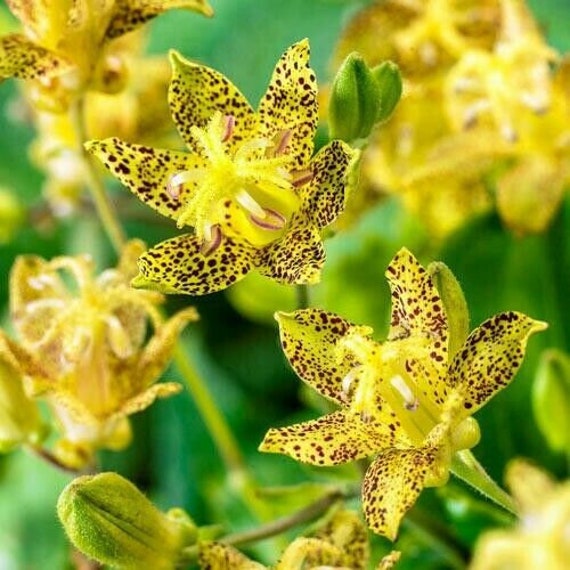A cluster of vibrant yellow orchids adorned with distinctive black spots and delicate purple pistils emerging from their centers, accompanied by bright yellow pistils, stands prominently in the foreground. Their lush green stems support several unopened buds, hinting at the promise of more blooms. Commonly known as "leopard orchids" due to their striking spotted pattern, these cheerful flowers create a captivating visual against a softly blurred backdrop, emphasizing the intricate details and colors of the orchids. The macro photography composition beautifully captures the lively interplay of yellow, black, purple, and green, resulting in an exquisite and joyful image.